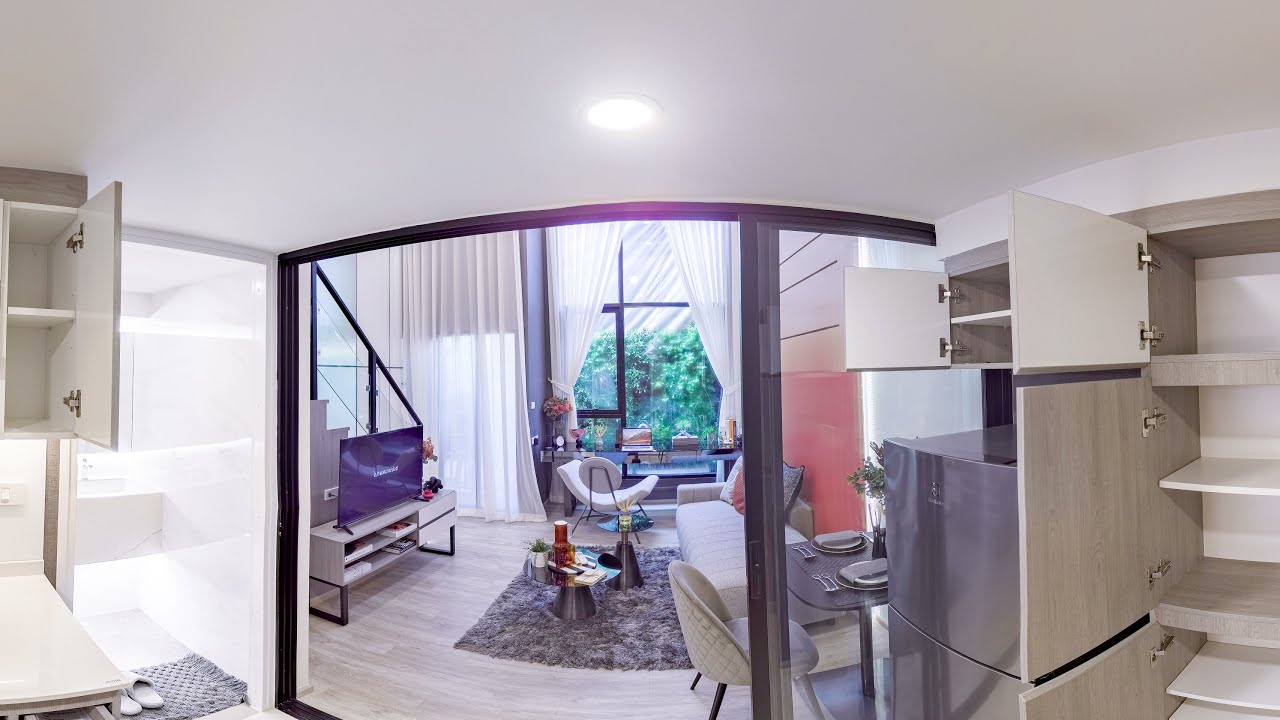The image captures an inviting indoor scene, looking from one room into the next within a home. The foreground features a room with a light-colored ceiling illuminated by a central light. On both the left and right sides of this room are open cabinets, accompanied by a stainless steel refrigerator on the right. A gray rug with white slippers lies at the bottom left. Centered in the image is a semicircular sliding glass door leading to an adjacent living area.

In the neighboring room, to the right, there is a cozy seating area with a lounging couch and a small chair placed opposite it. Along the left wall, a TV sits on a stand close to a table adorned with plates and silverware. The room is furnished with hardwood floors and a small rug, creating a warm ambiance. A staircase is visible in the background, ascending to the left. Floor-to-ceiling glass windows with black frames by the far side of the room are adorned with sheer white curtains, offering a view of green trees outside. A doorway leading to a terrace is also visible, enhancing the open, airy feel of the space.